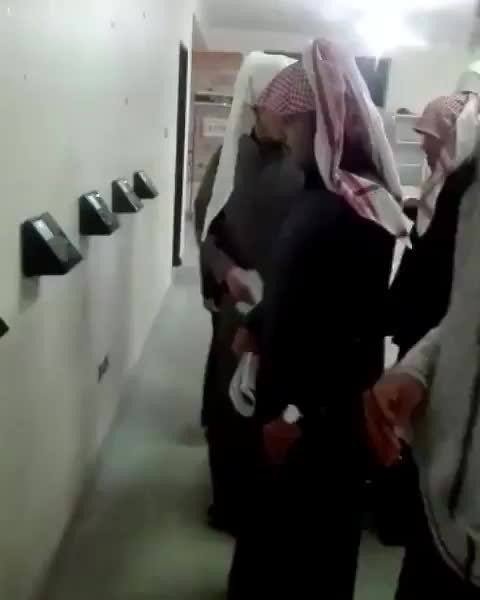In the photograph, several Arab men are gathered around triangular-shaped terminals mounted to a white wall at chest level. These terminals, which resemble pay stations or ATMs, are fixed securely and are drawing the attention of the men. They are wearing long, black robes and differing styles of headdresses; some men are adorned with red and white checkered headdresses while others wear solid white ones. The setting reveals a spacious room with a white floor and minimal visible decor. One man stands out, wearing a watch on his wrist. All the men seem to be focused intently on figuring out how to use the devices in front of them.